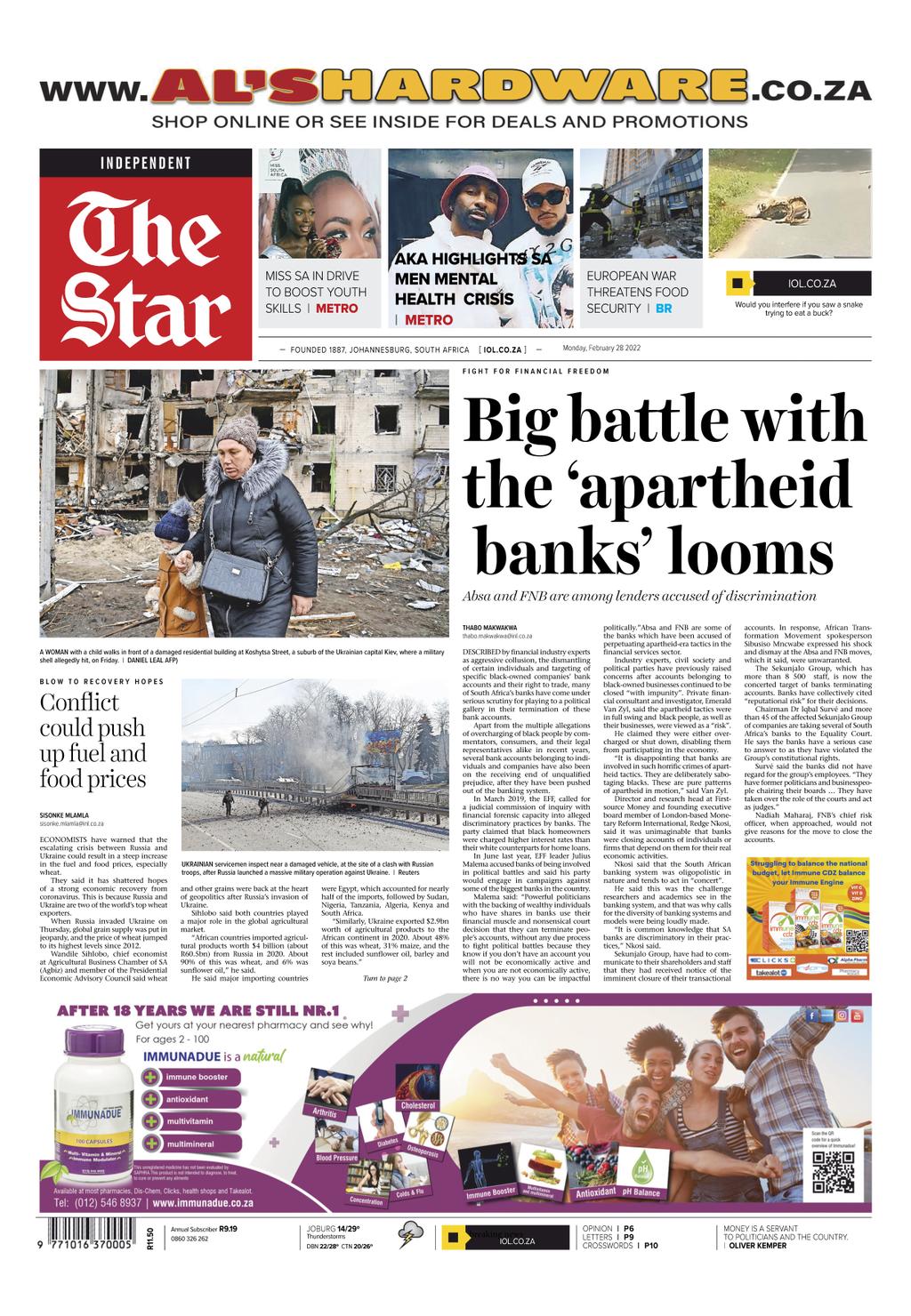At the top of the image, there is a banner featuring a website URL. The URL begins with "www." in black text, followed by "al's" in red, and then "hardware" in bold yellow block letters. This is followed by ".co.za" completing the web address. Below this banner, there is a section with the word "Independent" alongside a star icon inside a red square.

The image then transitions to a collage of different photographs. The first photograph features a woman adorned with a crown on her head. Adjacent to her, two men are pictured, both wearing hats and white shirts. Below these images, there is a picture of a woman carrying a purse, and donning a jacket, hat, and glasses. The background shows a building that appears to be in poor condition or damaged, possibly by a storm.

To the right, bold text reads, "Big Battle with the 'Apartheid Banks' Looms." Beneath this headline, another image depicts a scene in shades of gray, seemingly showing someone engaged in firefighting activities. To the left of this image, a caption warns, "Conflict Could Push Up Fuel and Food Prices."

Finally, at the bottom of the collage, there is an advertisement for a product that appears to be a medication or vitamin supplement. The bottle featured in the ad has a purple lid with the container itself being white, yellow, and purple in color.